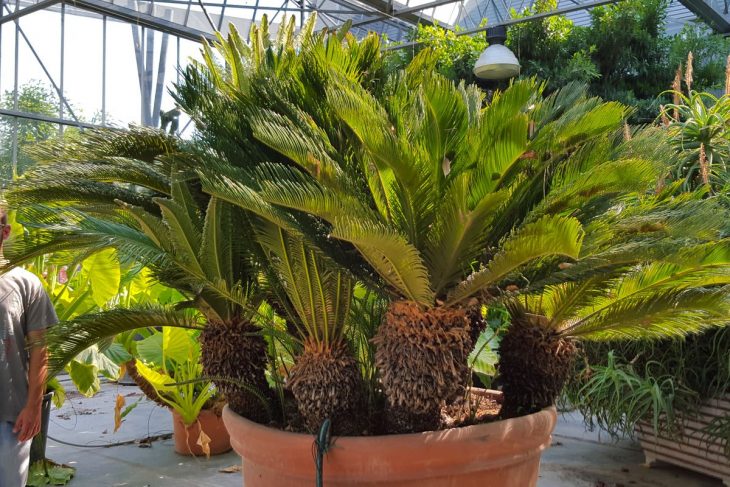The image captures a large, ornate plant housed in a terracotta pot, prominently positioned at the forefront within a glass and metal greenhouse. The plant features multiple trunks with brown, acorn-shaped bases from which lush, green leaves extend, resembling a fusion of palm and tropical fern leaves. The pot also includes a black hose. Above the plant, a clear bulb with a white base hangs from a black metal line, illuminating the scene. The greenhouse's glass walls and ceiling are visible in the background, showcasing several other plants and trees in both terracotta and wooden bases. To the left of the central plant, half of a man wearing a gray t-shirt and jeans is visible, partially cut off by the edge of the image. The ground appears to be cement, adding to the greenhouse's utilitarian aesthetic.